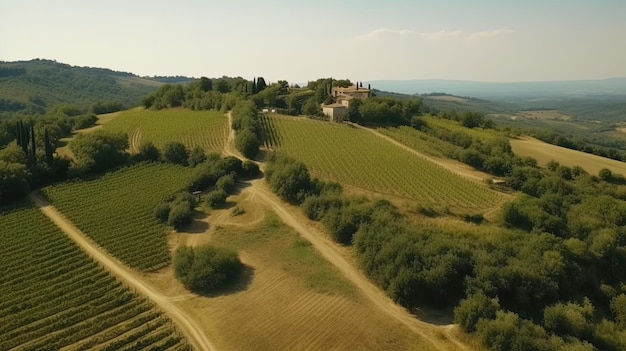This aerial landscape photograph captures a sprawling, lush green valley primarily composed of neat, rectangular fields arranged in rows, interspersed with well-maintained dirt tracks. The fields, possibly part of an extensive orchard, stretch out in an orderly fashion with clusters and rows of trees scattered throughout. On the lower right to middle right of the image, dense clusters of vibrant green trees stand out. Towards the center, slightly to the upper right, you can spot a group of brown or beige buildings with dark roofs, resembling old large houses but too distant for clear details. These buildings are nestled among trees at the base of a hill. Encompassing the valley are majestic, tree-covered hills or possibly low mountains, contributing to a picturesque background. The sky above is a pale blue adorned with some wispy white clouds, adding to the serene and timeless ambiance of the landscape.